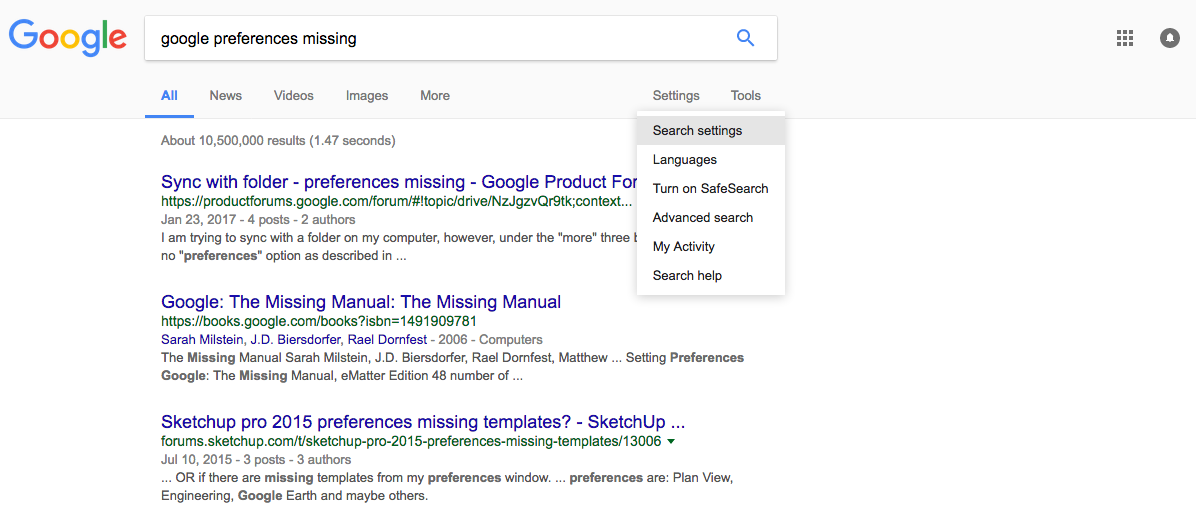The image is a screenshot of a Google search results page. At the top, the recognizable Google logo is displayed alongside the search query input in the bar, which reads "Google preferences missing." Directly beneath the search bar, there are categories labeled as "All," "News," "Videos," "Images," and "More." To the right, you notice sections titled "Settings" and "Tools." The "Settings" button has been clicked, revealing a drop-down menu that includes options such as "Search settings," "Languages," "Turn on SafeSearch," "Advanced search," "My Activity," and "Search Help."

The page indicates that approximately 10,500,000 results were found in 1.47 seconds. Three search results are prominently displayed:

1. **Google Product Forums: Sync with Folder - Preferences Missing**  
   - This result appears to be a thread in the Google product forums where a user discusses an issue related to syncing with a folder on their computer, noting the absence of a preferences option.

2. **Google: The Missing Manual, by Sarah Milstein, J.D. Bierstorfer, and Ryle Dornfest**  
   - This link points to a book titled "Google: The Missing Manual," authored by Sarah Milstein, J.D. Bierstorfer, and Ryle Dornfest. The book is seemingly unrelated to the search term.

3. **SketchUp Pro 2015: Preferences Missing Templates**  
   - The final result refers to a forum or support page for SketchUp Pro 2015, addressing an issue where preferences for templates appear to be missing.

Notably, the displayed results are not closely related to the original query about missing Google preferences, highlighting a potential discrepancy in the search algorithm's relevance.